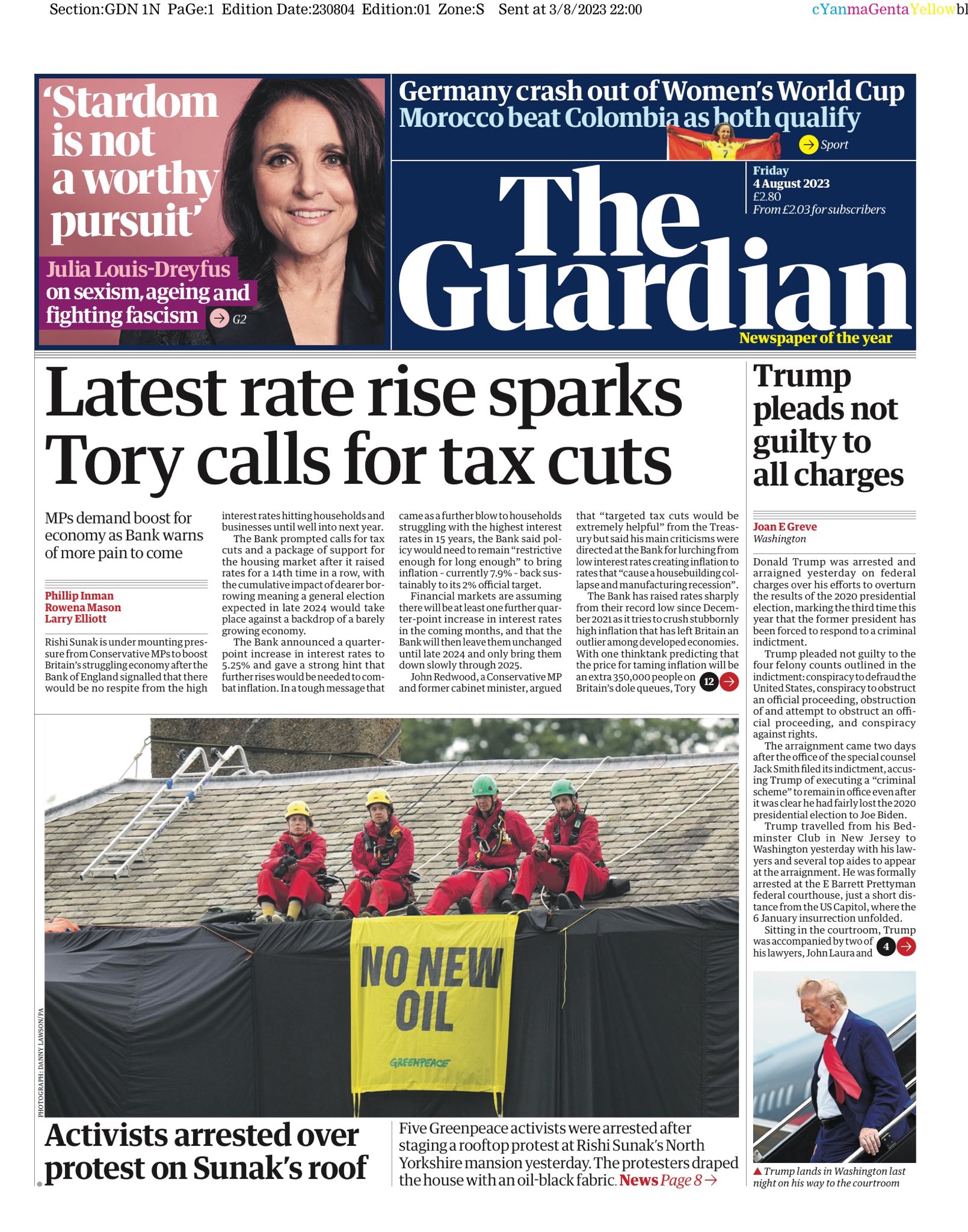**Detailed Caption for a Website Screenshot:**

The screenshot captures the layout of a website styled to resemble a traditional newspaper, filled with a dense amount of text and images. 

### Header Section:
- **Top Bar:** A white bar spans across the top, featuring black text indicating the section and edition details. It reads, "Section GDN," "Page 1," "Edition Date," and some numbers that appear to be "20004." Additional details include "Edition Zone" and a timestamp referring to "June 20, 2023, 22:00 hours."
- **Colorful Text:** To the right of these main details, there's a strip of text in varying colors such as blue, purple, and yellow. The text is not distinctly readable but begins with "eon."

### Main Content:
#### Left Section:
- **Profile Picture:** A square section contains a portrait of an older woman with black hair, smiling. 
- **Headline & Subheading:** To the left of her image is the text, "Stardom is not a worthy pursuit," followed by a subheading, "Julia Louis-Dreyfus on sexism, aging, and fighting fascism."
- **Background & Icon:** This section has a pink background with an arrow icon encouraging readers to explore more.

#### Middle Section:
- **Sports Headline:** The top row of the middle section states, "Germany crash out of Women's World Cup, Morocco beat Colombia as both qualify," accompanied by a small image of a soccer player with extended arms. A yellow circle with a blue arrow points to further reading.
- **Website Title:** Below the sports news, the title of the website, "The Guardian," is prominently displayed with a yellow subtitle reading "Newspaper of the Year" under the "IAN" of "Guardian."

#### Central Content Area:
- **Main Article:** The central content features a large headline, "Latest rate rise sparks Tory calls for tax cuts." Below this, there are four columns of tiny text providing details. The subheading reads, "MPs demand boost for economy as bank warns of more pain to come," followed by dark pink text that's difficult to decipher. Icons feature at the end of the article: a white "V" inside a black circle and a white arrow in a dark red circle.
- **Protest Image:** An image below shows four workers in red uniforms with helmets. The two on the left wear yellow helmets, while the two on the right have sea-green helmets. They're seated on a black-covered object with a yellow banner behind them reading, "No New Oil." A roof with a ladder is visible in the backdrop. The accompanying text above the image indicates, "Activists arrested over a protest on Sun X's roof," with a preview leading to page 8.

#### Right Sidebar:
- **Trump Article:** A smaller sidebar headline announces, "Trump pleads not guilty to all charges," accompanied by a small image of Trump exiting an airplane.

### Overall:
The entire content is set against a white background, segmented with clear visual and textual breaks resembling a newspaper layout, complete with headings, subheadings, images, and navigation icons for further reading.